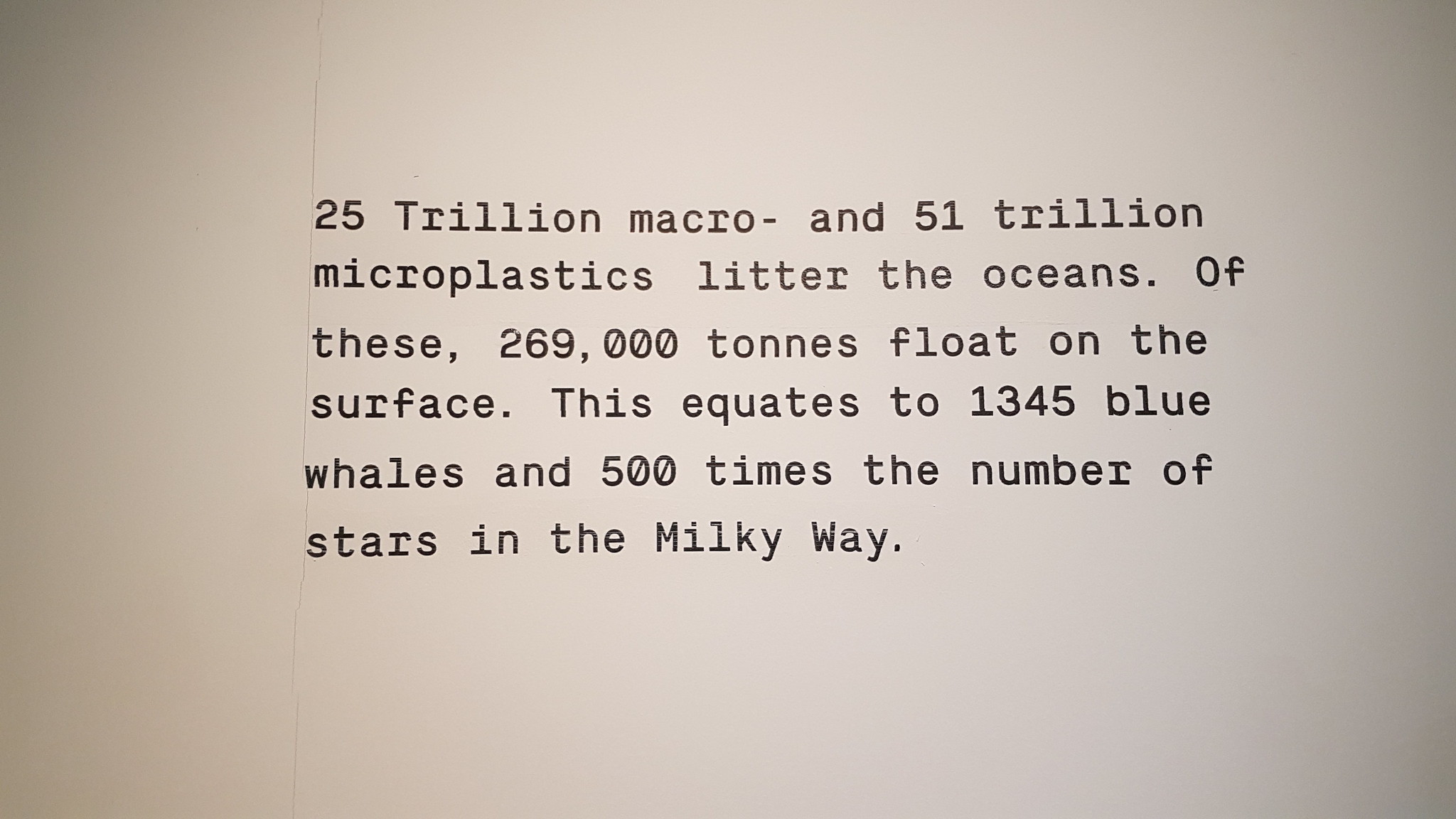The image is a close-up of a plain white piece of paper with a block of black text printed on it. The text reads: "25 trillion macro and 51 trillion microplastics litter the oceans. Of these, 269,000 tonnes float on the surface. This equates to 1,345 blue whales and 500 times the number of stars in the Milky Way." The text uses the British spelling "tonnes" and capitalizes the word "TRILLION." The rest of the page is blank, with a barely noticeable crease running down next to where the text starts, which could be a misprint or a faint pencil line. This detailed paragraph starkly highlights the staggering amount of plastics polluting the ocean, using impactful analogies to illustrate their vast quantities.